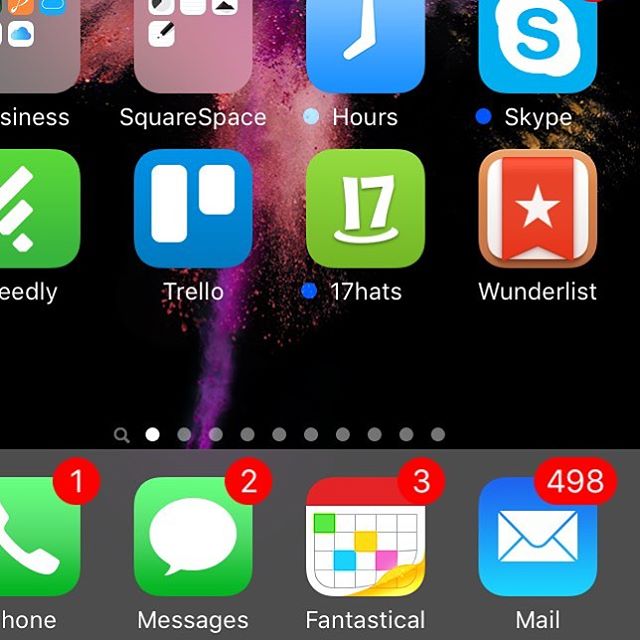This screenshot captures a partial view of a smartphone screen, with the top portion, including the battery percentage and service indicator, not visible. The screen displays a grid of eight different applications arranged in two rows. 

In the top left corner is a folder labeled "Business," containing several indistinguishable apps. To its right is another folder named "Squarespace," housing four apps. Next is the standalone app "Hours," followed by another individual app, "Skype."

On the second row, there is an app with partially visible letters "E-E-D-L-Y," possibly "Seedly" or "Feedly." This is followed by "Trello," "17 Hats," and "Wunderlist."

At the bottom of the screen are the primary applications: Phone, Messages, Camera, Fantastical, and Mail. Above these icons are several dots indicating the home screen pagination, with the first dot highlighted, signifying the current screen is the first of several.